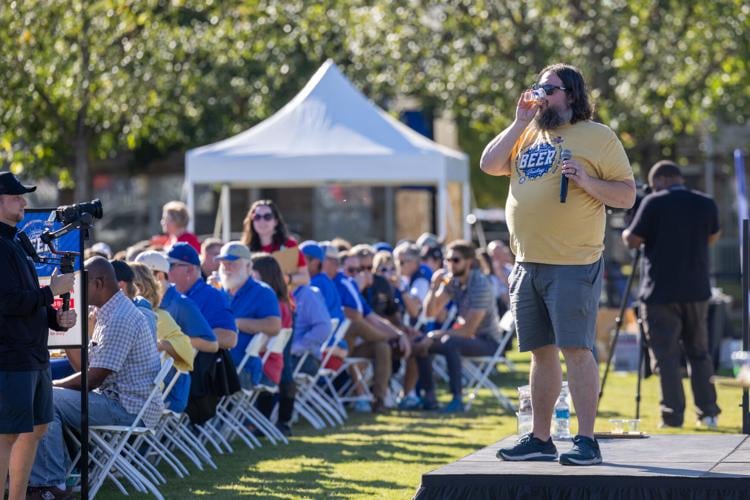The image captures a lively outdoor summer festival or reception set in a park with abundant green grass and deciduous trees. The focal point is a jovial man resembling Jack Black, standing on a black stage or podium. He sports a comical yellow t-shirt with the word "beer" emblazoned on it, knee-length dark gray shorts, and black sneakers. He has long hair, a beard, and wears sunglasses, enhancing his relaxed demeanor as he drinks beer from a plastic cup while holding a microphone. Nearby, several water bottles lie on the stage floor.

To the man's left, a cameraman in dark clothing, including a black hat and black shorts, captures the scene with a camera mounted on a tripod, aimed directly at him. In the background, a white gazebo tent further shades the area, and people sit on white folding chairs, their attention directed away from the main individual as they face another stage. Among the assembly, a woman in sunglasses stands, differing from the others who are seated. The scene is framed by a fine-mowed lawn, shadowed patches of grass, and buildings visible in the distance, perfectly capturing the essence of a sun-filled festival gathering.